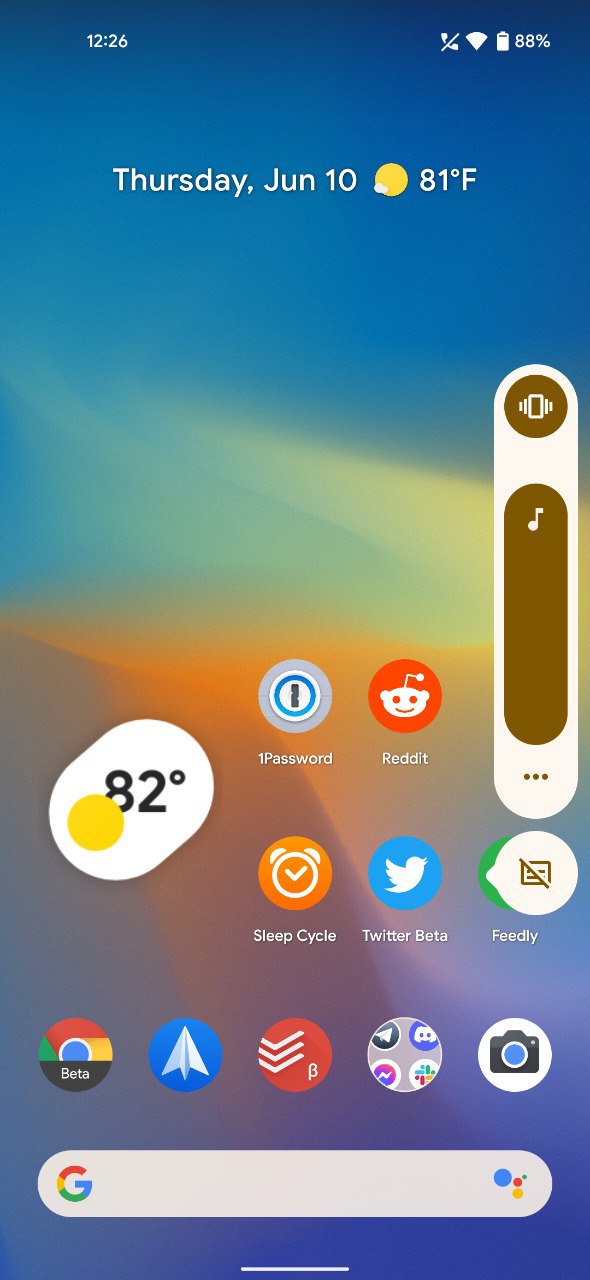The image appears to be a screenshot of a smartphone's home screen, showcasing a gradient background transitioning through various colors: from blue at the top, to a bluish-green, then yellow, followed by sandy orange, and finally a bluish-purple toward the bottom. 

On the top-left corner, the time is displayed in white as "12:26". Adjacent to this, there is a phone icon with a line through it, indicating that the phone is in "Do Not Disturb" mode. The Wi-Fi icon and battery icon are also present, with the battery level shown at 88%.

Directly beneath this status bar, the date and weather information are displayed. It reads "Thursday, June 10th," with a notation of "81 degrees Fahrenheit" and an icon suggesting slightly cloudy weather.

The screen contains several app icons arranged in rows. 

- The first row includes "1Password," and "Reddit," the latter characterized by its reddish background and a white, alien-like mascot.
- The second row features "SleepCycle" with an orange background, "Twitter" with a blue background, "Beta," and "Freely" with a green background.
- In the third row, there are the "Google" app, another "Beta" app indicated to be a likely new or test version of Google, an unidentified app with a red background and white downward arrows, and the "Camera" app. 

Overall, the layout is neatly organized with each app distinctly identifiable by its unique icon and background color.